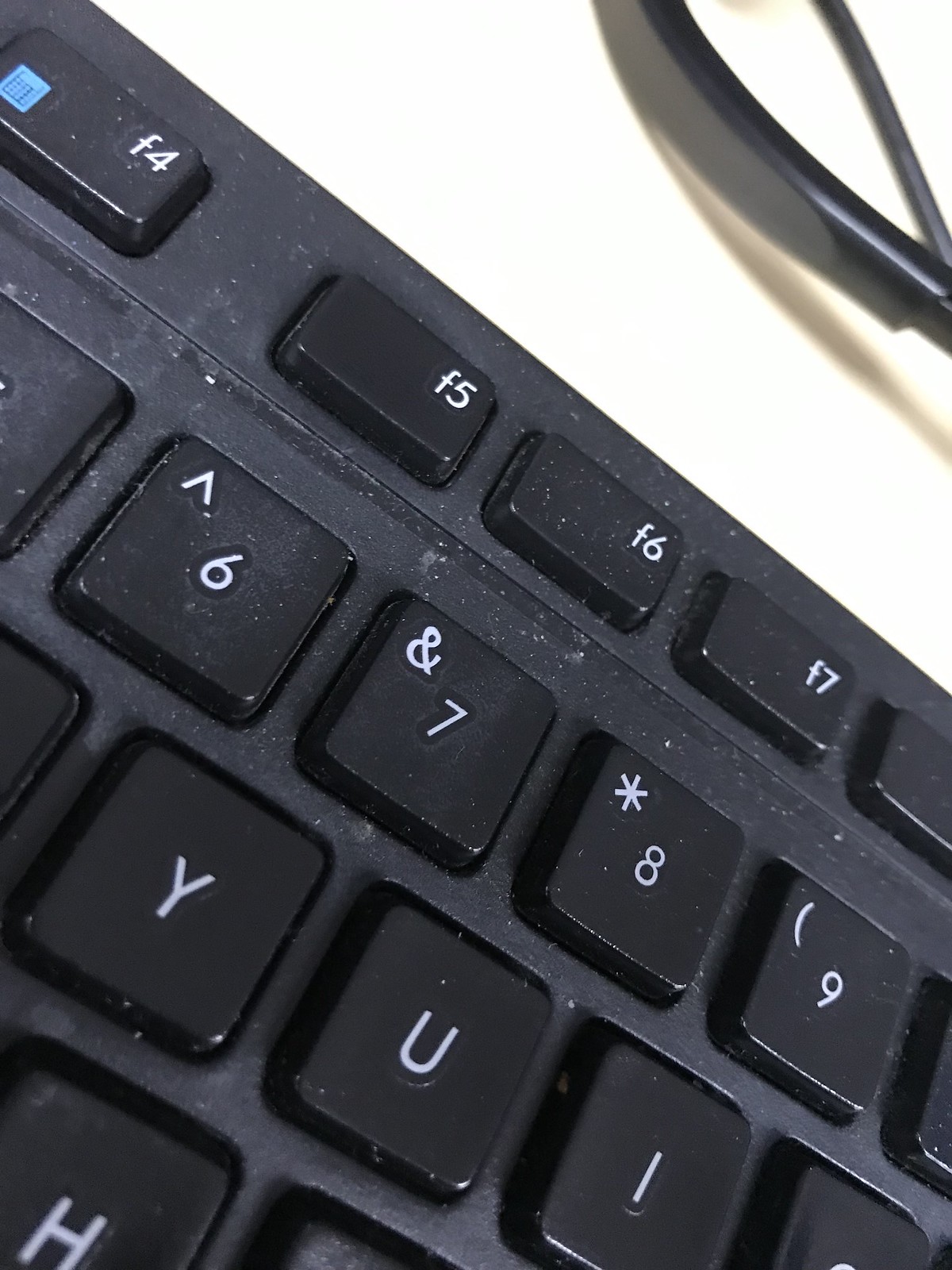This vertically-oriented color photograph captures a close-up, angled view of a partially visible black keyboard situated on a smooth, light-colored desk surface. The focal point is the bottom left part of the image, showcasing keys such as F4, F5, F6, F7, 6 with an up arrow, 7 with an ampersand, 8 with an asterisk, 9 with an open parenthesis, and the letters Y, U, I, and H. The keys are black with white text, all clearly readable without any fading. The keyboard itself shows signs of usage with visible dust and minor debris, including white flakes. In the top right corner, a black and white object, possibly part of an electrical cord or pair of glasses, is partially visible but out of focus. A shadow beneath this object hints at its raised position above the desk surface.